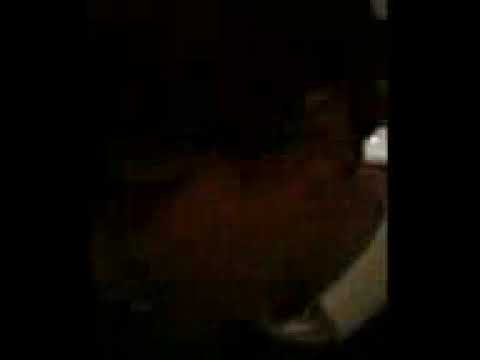This image is a dimly lit, color photograph in portrait orientation, set against a black rectangular background. At its center is a blurry, very close-up selfie of an individual whose gender is indeterminate due to the darkness and lack of clear features. The face, partially illuminated by a small bit of light on its left side, reveals faint outlines of eyes, a nose, and a small bit of dark hair. The person appears to have darker skin. Behind them, in the top left corner, there's a subtle glow from what might be a lamp, adding minimal backlighting. The person is dressed in a white collared shirt and a dark jacket. The image is framed by black rectangles on either side, enhancing the focus on the central, unclear visage, reinforcing the photographic representationalism realism style.